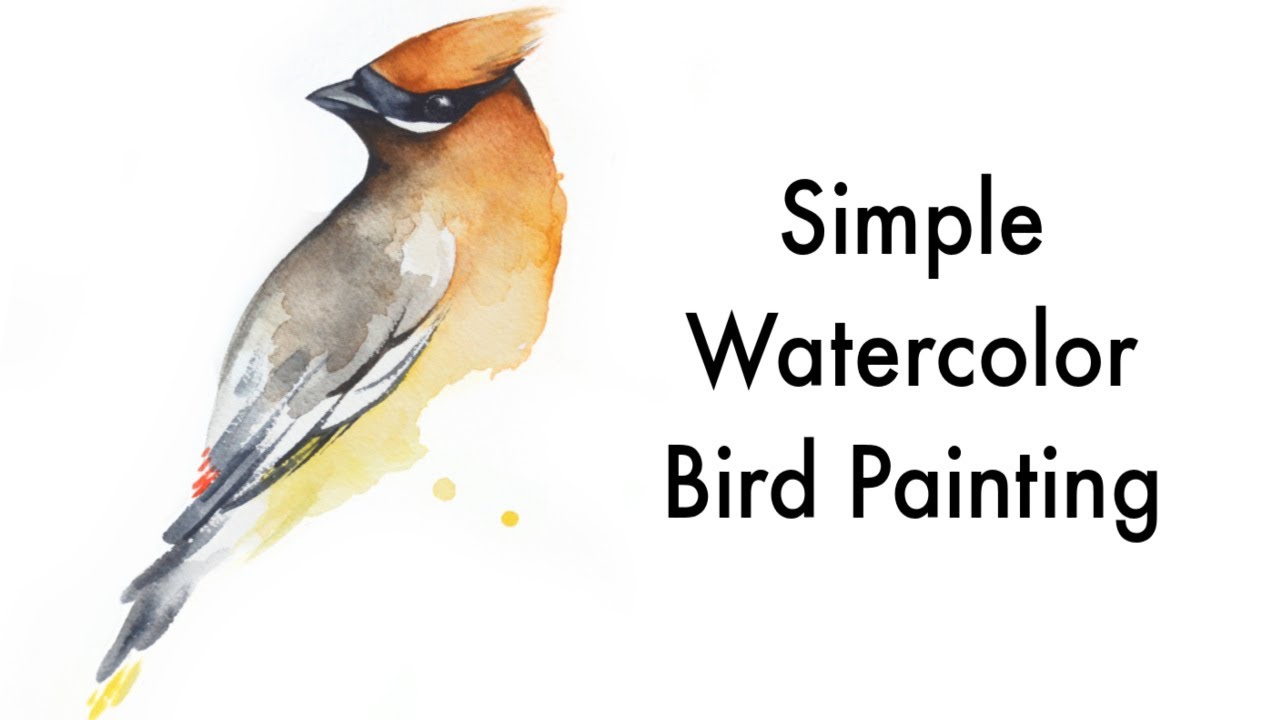The image features a detailed watercolor painting of a bird set against an all-white background. On the right side of the image, large sans-serif black text reads "simple watercolor bird painting." To the left of this text, the bird displays a rich ombre of colors: its head and upper body are a vibrant rust orange that seamlessly fades into a lighter yellow toward the underbelly. The bird's wings exhibit a complex blend of gray, white, black, brown, and lightly tinged red at the feather tips, with hints of yellow at the tail end. The bird's beak is gray with a small white spot, and its eyes are strikingly black with a black stripe reminiscent of a raccoon's mask. Below the bird's body, there are two small yellow dots, suggesting the eventual placement of legs. The overall composition is remarkably detailed for a watercolor, combining both warm and cool tones to create a lifelike representation.